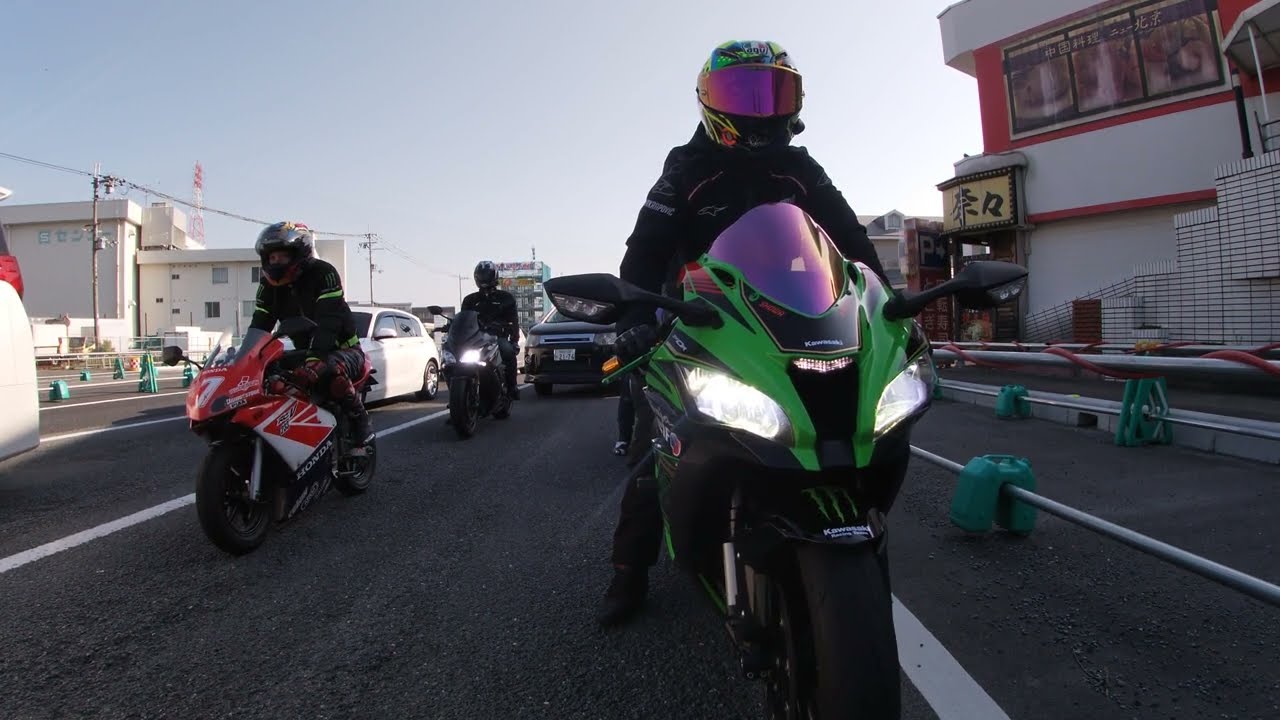In the image, we observe a motionless scene set on a road during a sunny day. Three motorcyclists dominate the foreground, all geared up in black outfits and helmets. The closest rider's motorcycle is a striking green and black with a purplish protective glass. The rider sports a distinctive white helmet splashed with vibrant rainbow colors and a visor shaded in pink and purple hues. To the left, another motorcyclist rides a red and white bike, wearing a similarly black outfit with hints of red and a silver helmet partially exposing their eyes. Further back, the third rider in black attire straddles a white motorcycle. Surrounding these riders, there are several cars, including a white van on the middle left and a white car slightly rightward in the background.

The backdrop features two prominent white buildings in the back left, one taller than the other, with power lines running diagonally overhead. On the right, a structure with a red-trimmed upper half stands out, accompanied by a yellow sign bearing Asian characters, specifically Chinese, written in black. The entire scene exudes a sense of stillness, despite the bustling potential of the road, captured vividly against the bright blue sky.